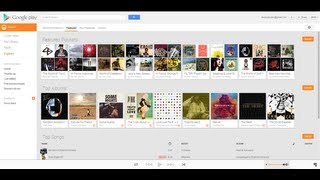In this image, we see a screenshot from the Google Play interface. The Google Play logo is prominently displayed in the upper left corner, accompanied by a search bar. In the upper right corner, there are at least three buttons, although they appear pixelated and difficult to read. 

The main section of the screen is dedicated to "Featured Playlists," which are represented by square thumbnails each consisting of four album covers arranged in a grid. Beneath these thumbnails, there are text labels likely indicating the titles of the playlists. 

Below the Featured Playlists, the next section is labeled "Top Albums." This section features individual album covers, including a noticeable pink cover, the album "Some Nights," and another cover by Justin Timberlake.

Further down, there is a section titled "Top Songs." The text and images in this section are quite small and pixelated, but two items are visible.

At the very bottom of the screen, the media controls are located. These include a play button, a forward button, and a backward button. On the lower right side, there is a volume bar, which is adjusted all the way to the maximum.